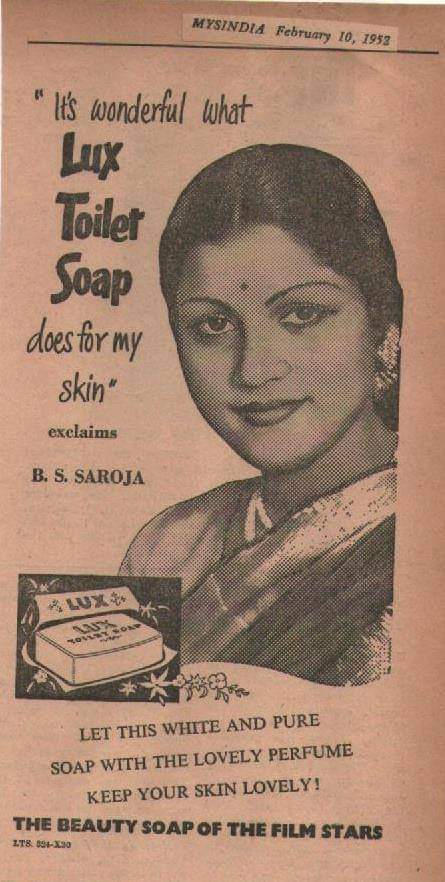In this vintage advertisement, dated February 10th, 1952, we see a classic promotion for Lux Toilet Soap. The image features an Indian woman, likely a film star, dressed in traditional attire and positioned centrally, gazing directly at the camera. The background is a muted pink hue, contrasting with the monochrome elements of the ad. At the top, it proudly announces "Miss India, February 10th, 1952," with a testimonial reading, "It's wonderful what Lux Toilet Soap does for my skin," exclaims B.S. Saroja. The ad emphasizes the soap's qualities, describing it as "white and pure soap with the lovely perfume" that "keeps your skin lovely," branded as "the beauty soap of the film stars."

In the bottom left of the image, a bar of Lux soap is depicted emerging from its box, accompanied by small white flowers, symbolizing its purity and gentle fragrance. The advertisement, with its half-tone black and white print, reminiscent of old newspaper styles, pitches the soap as a premium choice for those aspiring to the glamor and beauty of film stars.